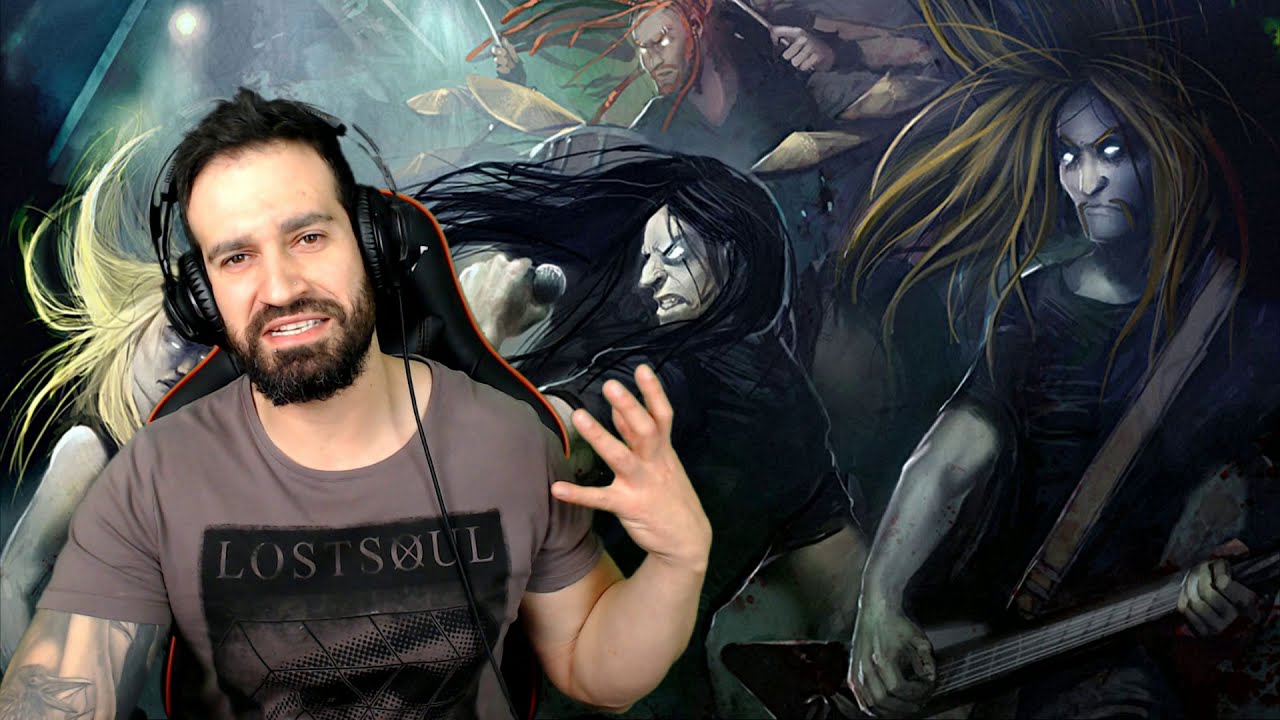The image captures a man in his mid-30s with a beard and dark hair, sitting in a black and red gamer chair. He is wearing over-ear black headphones connected by a visible cable and a brown t-shirt with a black square featuring the text "Lost Soul," with the 'O' crossed out. His right arm displays tattoos, and his left hand is raised near shoulder height, gesturing as if expressing a point mid-conversation. The background is vividly illustrated with a mural depicting a heavy metal band, where the band members have exaggerated features like glowing white eyes and animated movements. The mural shows, from left to right, a blonde-haired musician (instrument unclear), a microphone-wielding vocalist with black hair, a wild brown-haired guitarist, and a red-haired drummer. This detailed scene suggests he might be streaming or involved in a podcast likely focused on metal music, given the thematic consistency of his attire and the backdrop.